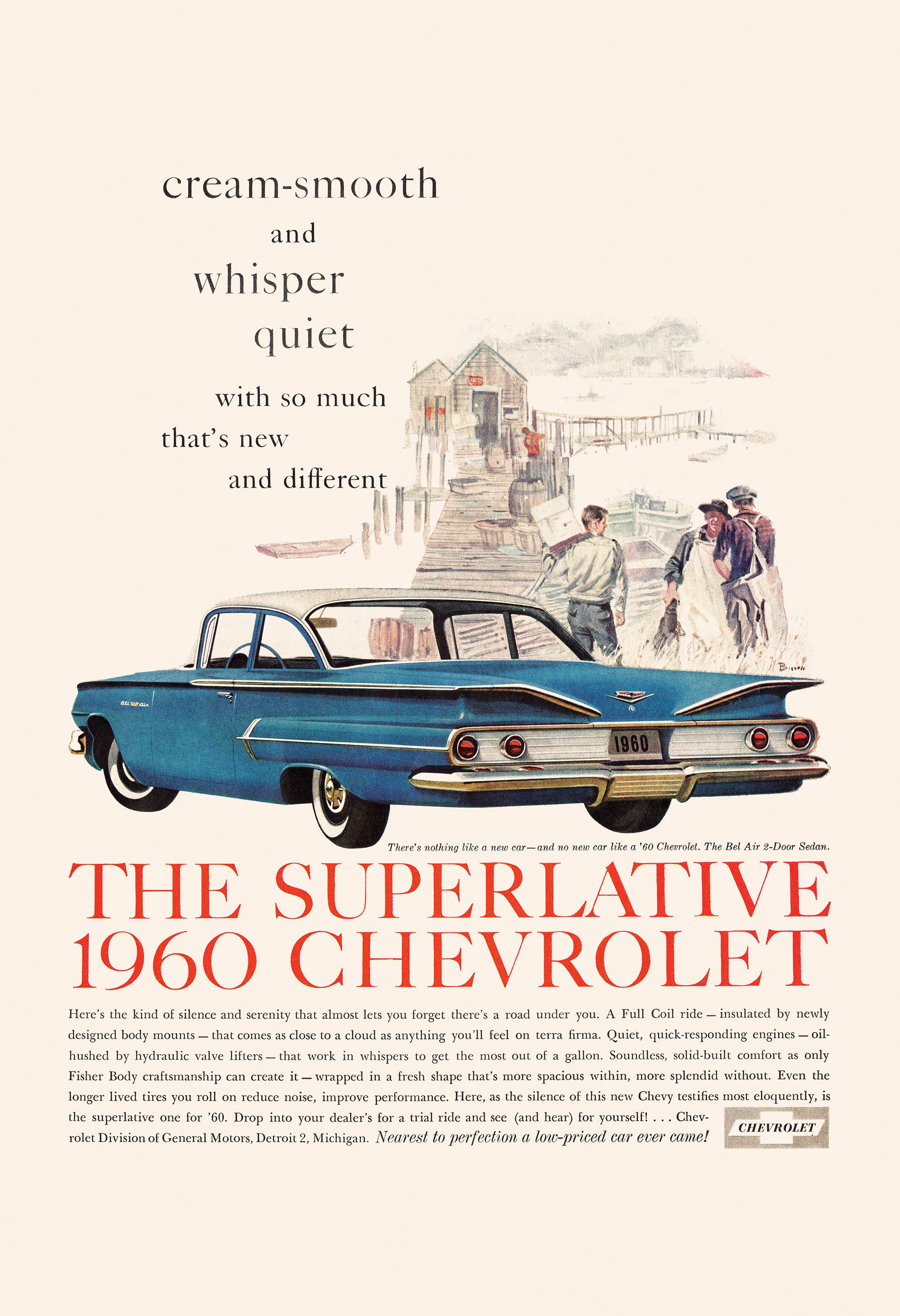This vintage-style advertisement, seemingly from a magazine, prominently showcases the rear view of a classic 1960 Chevrolet in vibrant blue with a white top, set against a cream background. Above the car, bold text announces, "Cream smooth and whisper quiet, with so much that's new and different." Below the image, red text proclaims it as "The Superlative 1960 Chevrolet." Illustrated in the backdrop are lively scenes of people enjoying activities on what appears to be a pier, with various boats and a bridge in the distance, enhancing the car's perceived versatility and appeal as both a practical family vehicle and one for leisure and fun. The ad also contains a detailed paragraph extolling the vehicle's quietness, fuel efficiency, and robust build quality, all underscored by the iconic Chevrolet symbol at the bottom.